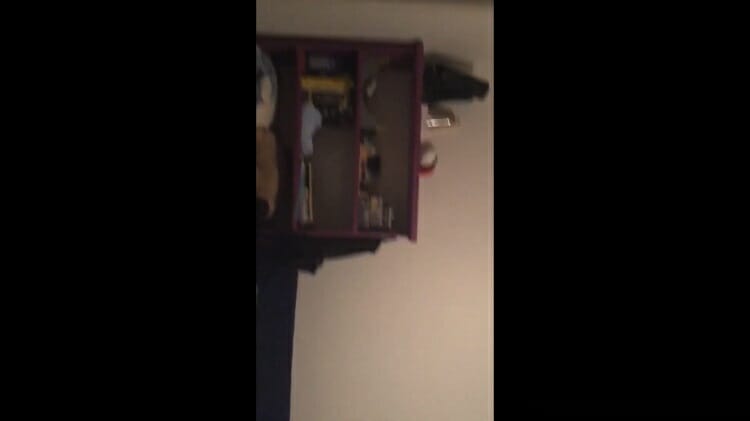The image depicts an off-white wall flanked by black sections on the left and right. At the center, a red shelving unit with red shelves and a brown backing stands prominently. On the top left shelf, there is a black cube or square. The second shelf houses some books, several of which stand upright with black and yellow spines, alongside thinner publications that resemble magazines with white lines. The bottom shelf contains miscellaneous items, possibly including a white cushion with blue accents on the left and a light brown cushion on the right. The photo is quite fuzzy, making some details hard to discern. Additionally, a shadow cast by a light fixture falls on the right side of the wall, partially obscuring the bookshelf.